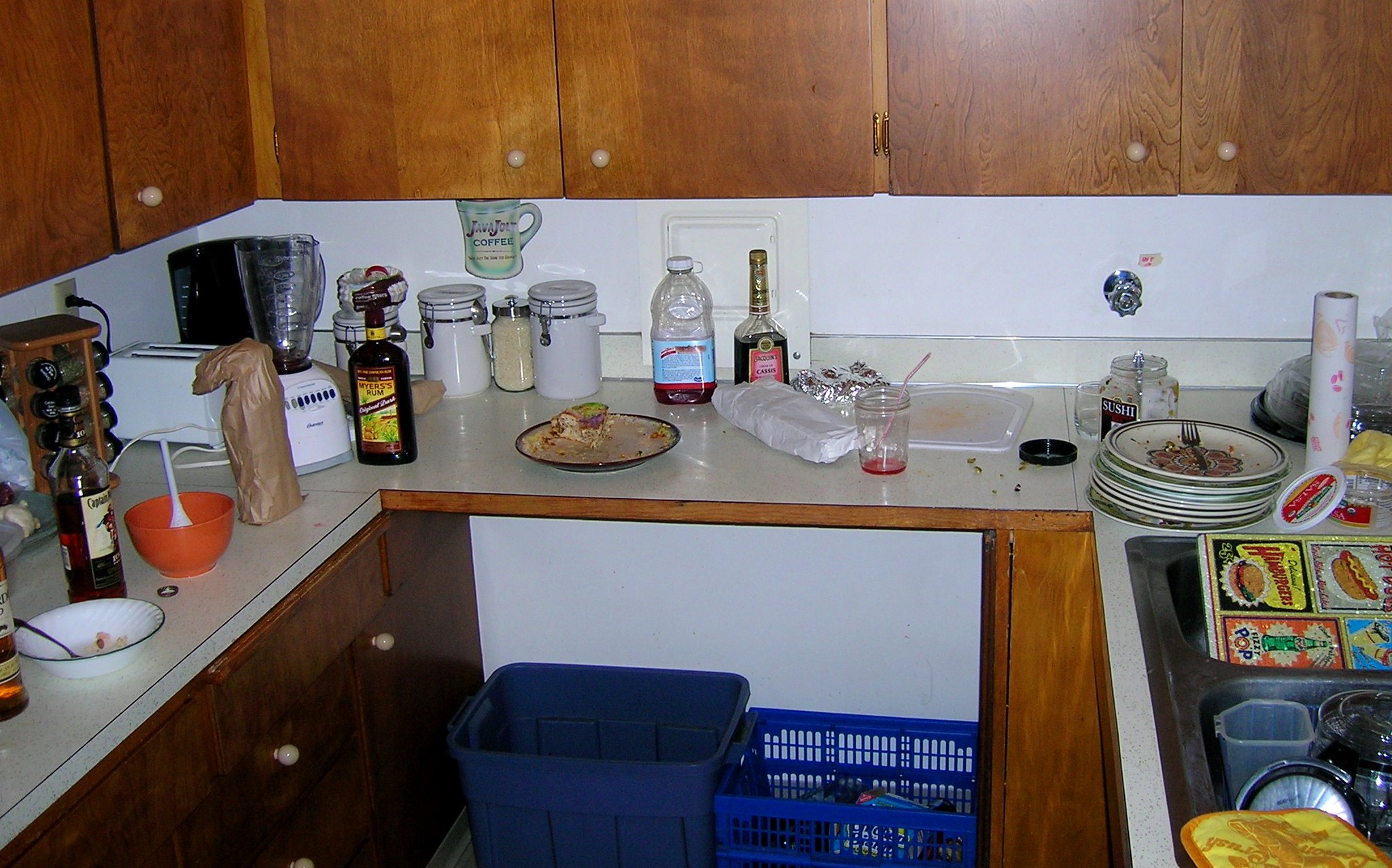The close-up image captures a section of a cluttered kitchen with a U-style arrangement. Dominating the scene are brown cabinets topped with white countertops that appear to be made of either tiles or Formica. The white wall behind the countertops further accentuates the untidy state of the kitchen. Plates with food particles are scattered across the countertop, contributing to the disarray. 

In the upper to middle right corner, a stack of dirty plates, one with a fork in it, adds to the chaotic atmosphere. The lower right corner reveals an overflowing sink brimming with more unwashed dishes. On the left side, two bottles of wine stand amid additional dirty plates and bowls, further highlighting the kitchen's unkempt condition.